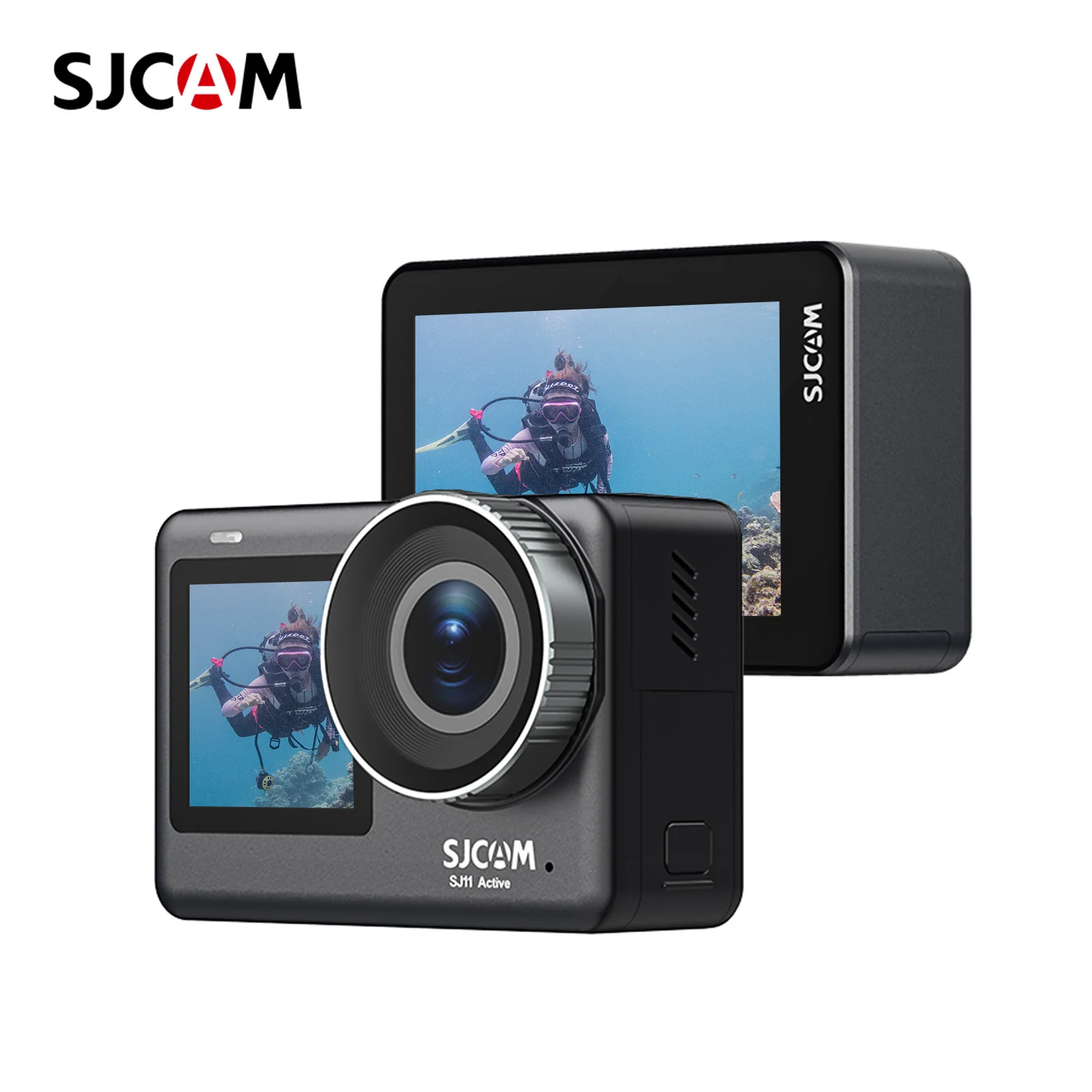This is a detailed advertising color photograph of the SJCAM SJ11 Active camera showcasing both its front and back angles. The camera itself is predominantly black with some dark gray accents, featuring a large, wide lens that occupies about half of its front surface area. Just below the lens, the brand name "SJCAM" is prominently displayed, with the distinctive "A" outlined differently. Beneath this branding, the model name "SJ11ACTIV" is visible.

To the left of the front lens, there's a smaller screen depicting an underwater scene where a woman is scuba diving among coral, wearing pink goggles and yellow flippers. The same image is duplicated on the larger screen on the back of the camera, emphasizing the camera's action-oriented capabilities. The SJCAM branding appears again on the back right side of the camera. Additionally, the top left corner of the advertisement features the SJCAM logo in black letters with the "A" encircled in red and displayed in white, reinforcing the brand identity.